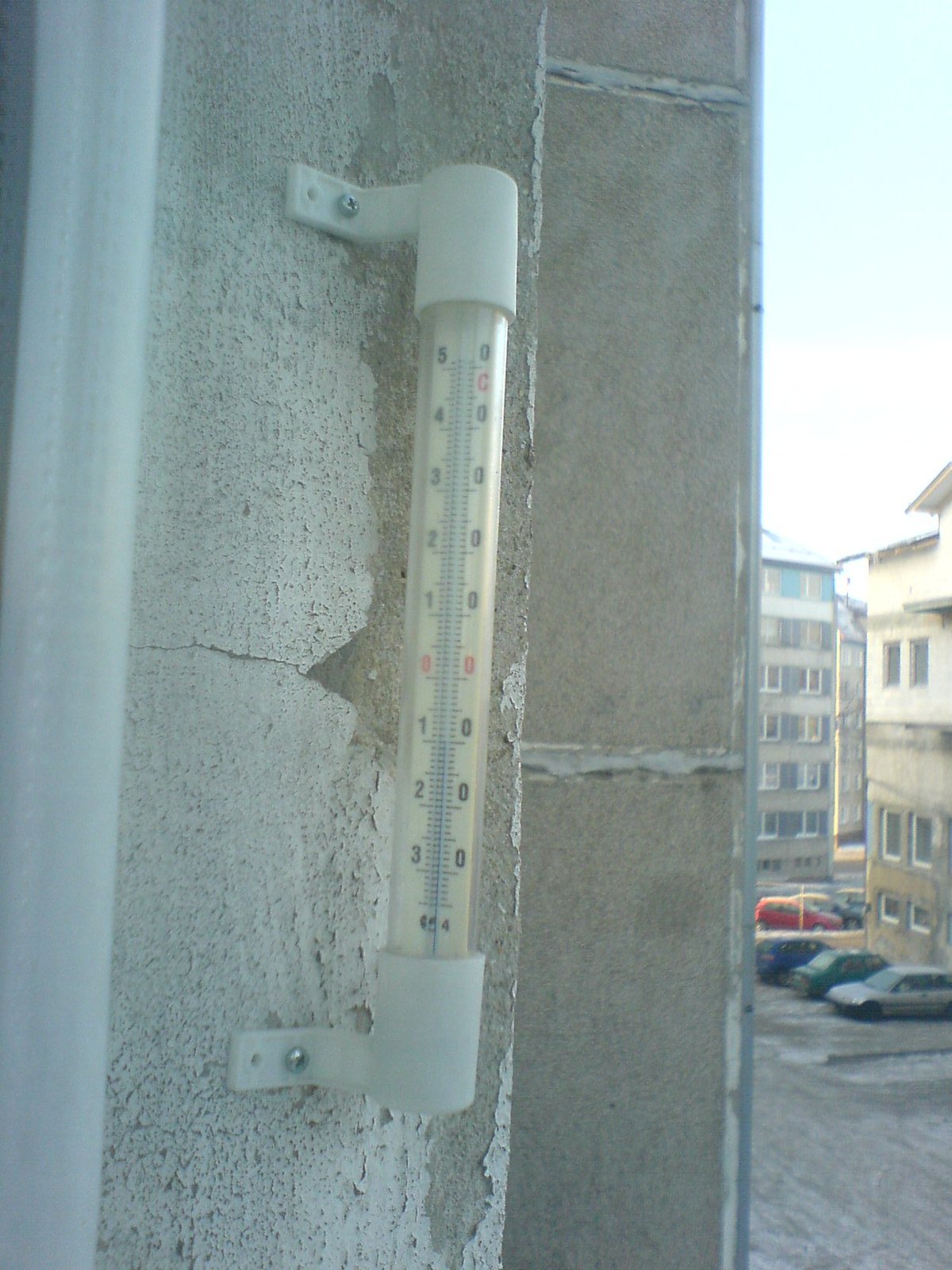On the left side of the image, occupying approximately three-fourths of the frame, there is a prominent concrete wall. Attached to this wall is a detailed thermometer, which is secured with two white brackets at either end. The thermometer is clear, displaying both Fahrenheit and Celsius scales, with red zeros marked in the center indicating the current temperature.

On the right-hand side of the image, in the remaining quarter of the frame, there are two concrete buildings—a three or four-story house and a five-story house—along with a busy parking lot. The parking lot is filled with a variety of cars in different colors and styles, including a gray, green, blue, red, and black car. The scene is vivid and detailed, providing a snapshot of an urban environment with contrasting elements of architecture and transportation.